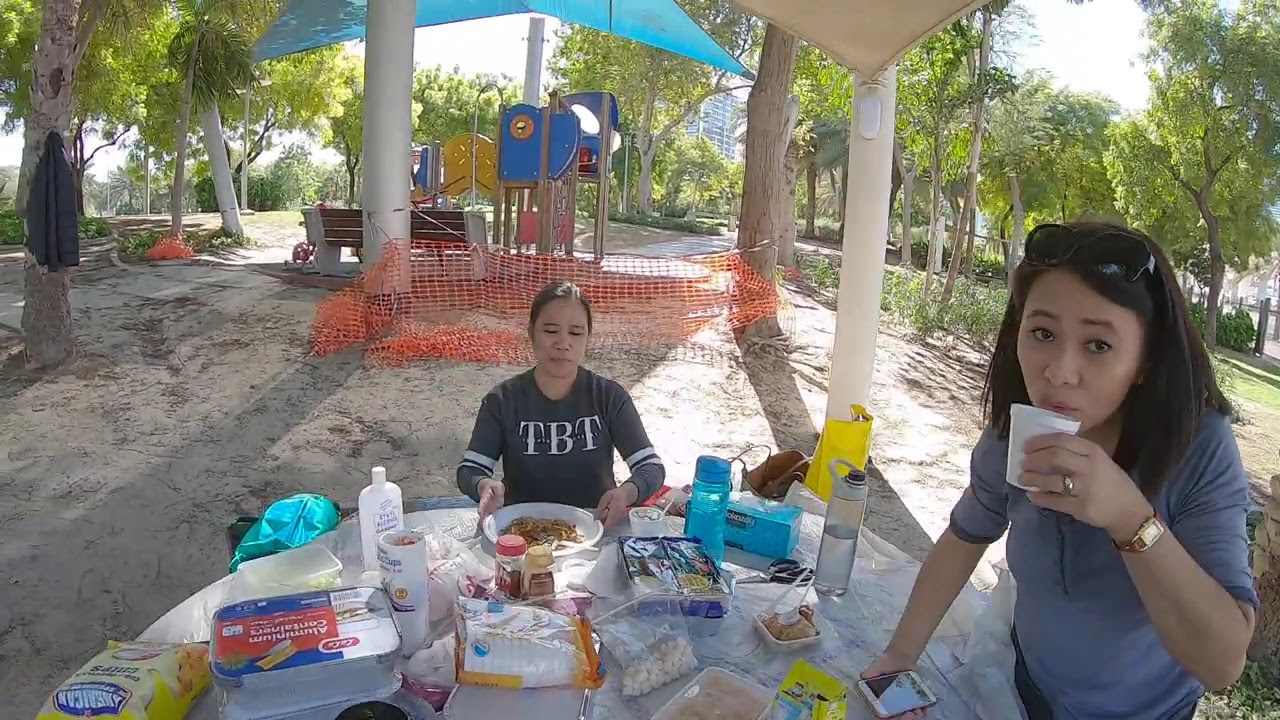Two dark-haired Asian women are enjoying a meal outdoors at a round, white table covered with various foods, containers, bags, and cups. The woman in the center is facing the camera directly, wearing a navy blue, long-sleeved t-shirt with "TBT" printed on it, and has a plate in front of her. To her right, the other woman is wearing a plain blue t-shirt with sunglasses on her head, drinking from a white cup. The table, which seems to be either marble or plastic, is laden with a generous spread, including water bottles and possibly deli meats and chips. The background features palm-like trees, a bench, and multiple colorful playground structures. There are also umbrellas providing shade and an orange barricade netting positioned between two trees, suggesting a park-like setting.